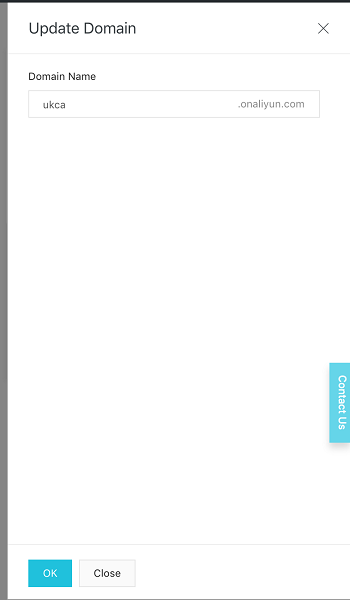The website features a sparse, minimalistic design with a predominantly dark theme. On the left side and the top, there are black outlines, with the left side being notably thicker than the top. At the top left corner, the text "Update Domain" is displayed, adjacent to an 'X' button on the far right.

Beneath this heading, a section labeled "Domain Name" is present, featuring a text input box where users can enter their domain name. In this instance, "UKCA" has been entered, and next to the input box, the domain extension "onal.yun.com" is automatically filled in.

On the right side of the page, a vertical turquoise-colored box labeled "Contact Us" is prominently displayed, providing users with a conspicuous call to action.

At the very bottom of the page, a light gray line spans the entire width. Just below this line, there are two buttons. The first button is teal-colored with the text "Okay," followed by a very light gray-colored button labeled "Close." These elements mark the conclusion of the webpage's content.